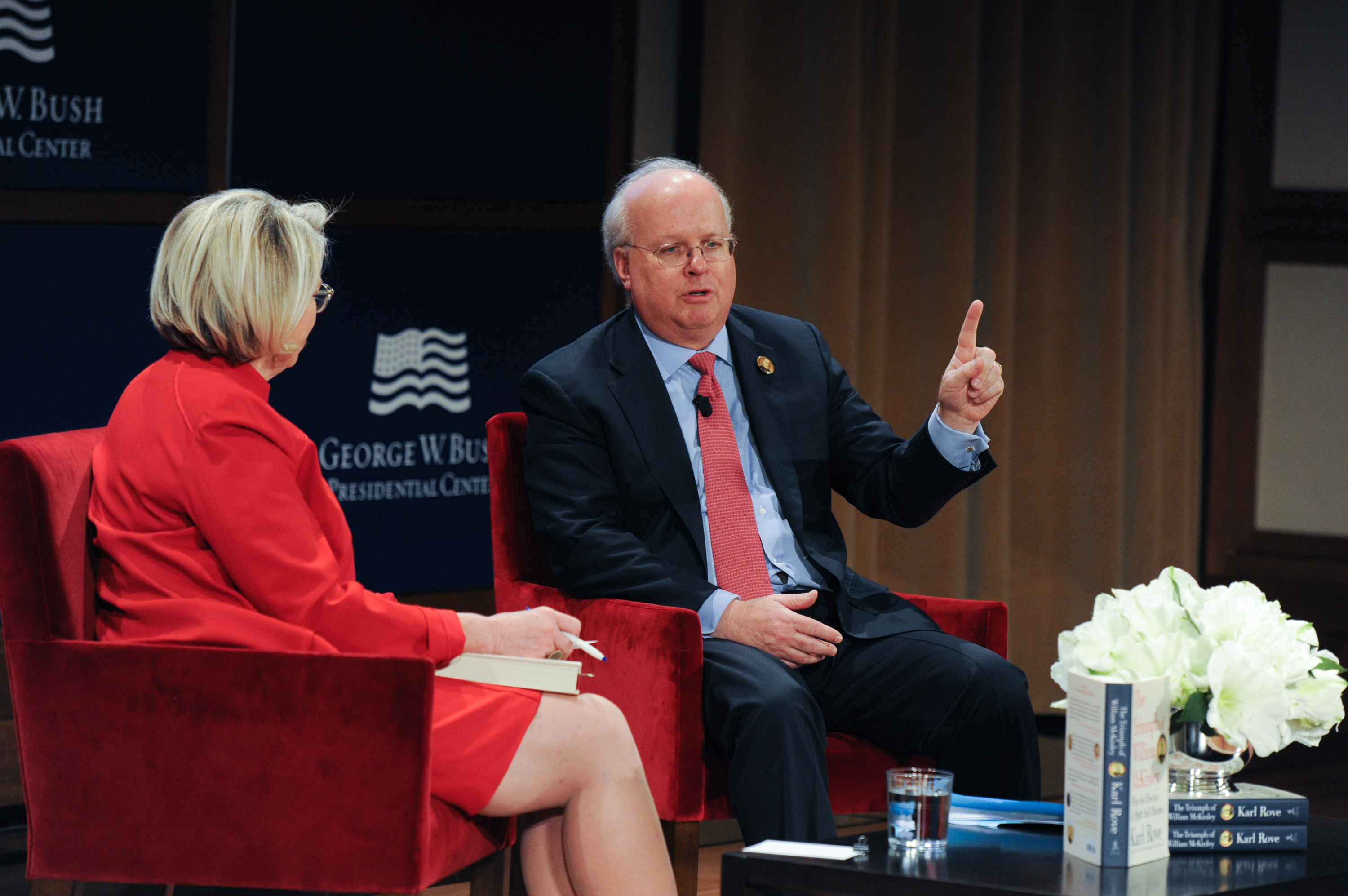The photograph features Karl Rove seated in a red velvet chair, dressed in a dark blue suit, blue shirt, and a red tie, with glasses perched on his face and a black microphone clipped to his tie. He has similar colored pants to his jacket. Rove is mid-speech, gesturing with his left hand, index finger pointing upwards, emphasizing a point. Next to him, a woman, likely the interviewer, is seated in another red chair. She is wearing a red dress, holding a pen and some papers in her lap, and looking attentively at Rove. The setting is the George W. Bush Presidential Center, indicated by a blue banner with the center's name and an American flag logo in white lettering in the background. In front of them is a coffee table adorned with a display of Rove's book, a glass of water, and a small flower arrangement, contributing to the formal interview atmosphere.